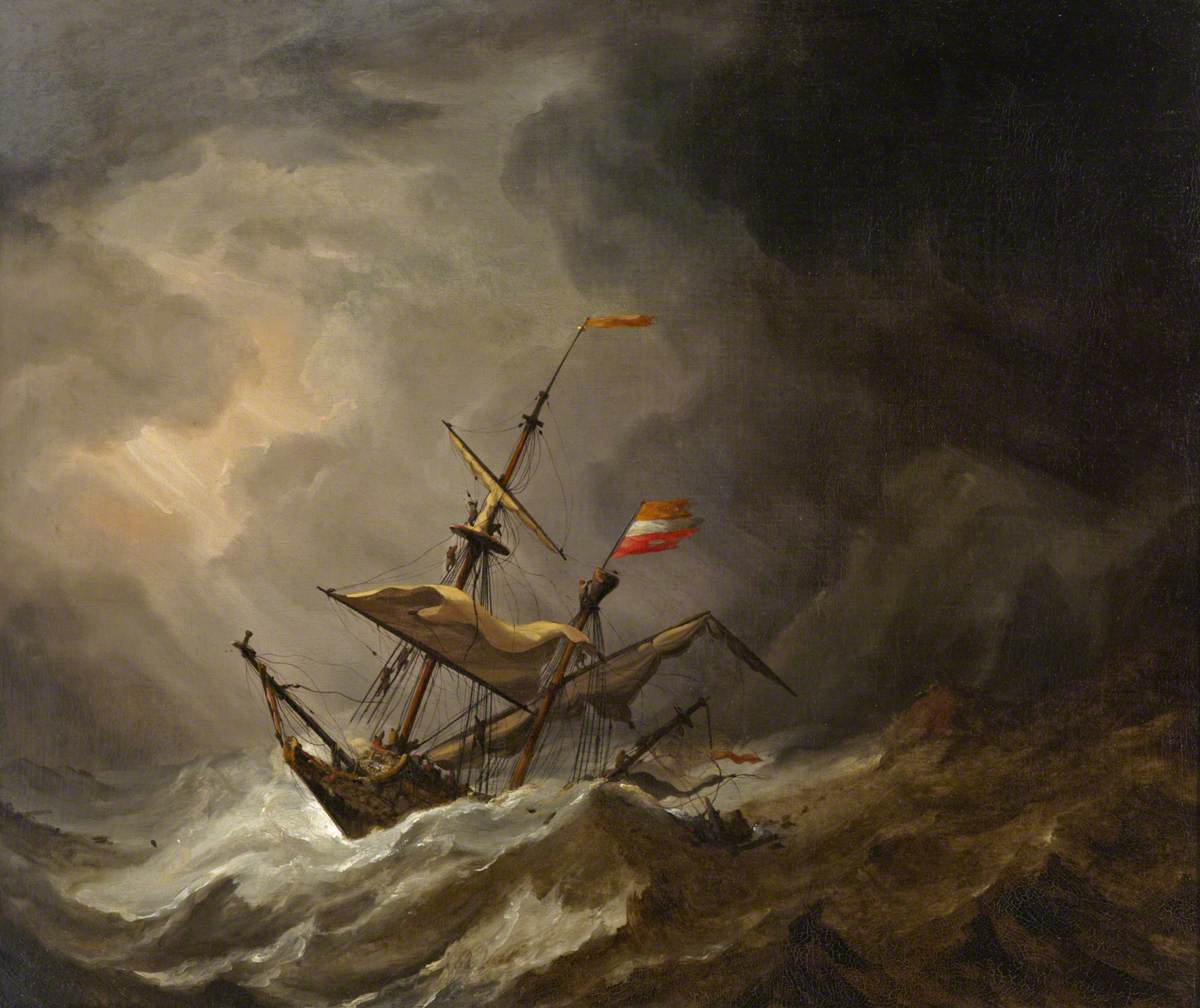This painting vividly captures a tumultuous sea scene featuring an old-time sailboat caught in a fierce storm. The majority of the water is rendered in dark, murky shades of brown and gray, with towering waves crashing around the vessel. The boat itself is prominently brown with multiple sails, many of which are tattered and torn from the relentless waves. It also bears a flag colored yellow, white, and red, though partly ripped, waving from the topmast. The ship is angled dramatically, with its front tipping upward, indicating its struggle against the powerful sea. The background is divided into darker, storm-laden skies on the right, and somewhat lighter, though still ominous, grays to the left. A small break in the clouds allows a sliver of sunlight to pierce through, casting an eerie light onto the beleaguered ship. The overall atmosphere is one of chaos and desperation, as the ship battles against the overwhelming forces of nature.